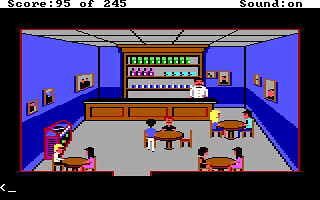This detailed screenshot from a vintage 80s or 90s video game showcases pixelated, simplistic graphics emblematic of 8-bit or even 4-bit design. The scene depicts the interior of a retro bar or soda shop with blue walls consisting of a lighter blue upper section and a darker blue lower section, adorned with pictures and portraits. The ceiling is grey, and grey panels accent the shop's structure. In the center of the room are four circular brown tables, each surrounded by seated patrons. Toward the left side of the room stands a pink and purple jukebox, adding a splash of color to the setting.

Dominating the right side is a tall wooden shelving unit with multiple shelves filled with a variety of colorful bottles—green, pink, blue, and light blue—likely containing liquor. In front of the shelves, a male bartender dressed in a white suit tends to the customers. Notably, the screenshot also features game interface details: the top left corner shows the score, which is 95 out of 245, while the top right corner indicates that the sound is on, both of these over a white background. The image is framed by a thick black border, followed by a red stripe edging the rectangular game display.